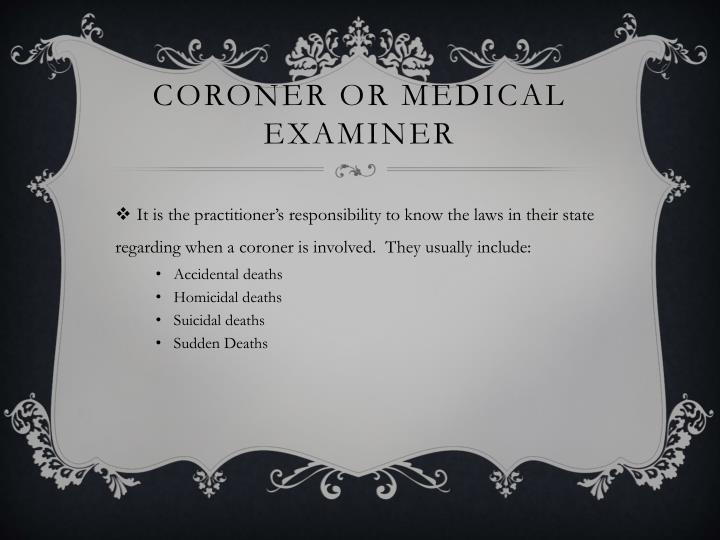This black and white image resembles a formal certificate featuring a detailed, decorative design. At the center, the top title reads "CORONER OR MEDICAL EXAMINER" in bold, capitalized black text. A light gray background graces the middle portion of the image, adorned with intricate, floral etchings and a decorative curly Q line separating the title from the body text. Below the title, the text states: "It is a practitioner's responsibility to know the laws in their state regarding when a coroner is involved." Following this statement, a list of four bullet points highlights specific instances requiring a coroner's involvement: accidental deaths, homicidal deaths, suicidal deaths, and SUDDEN DEATHS (with the latter term fully capitalized for emphasis). The image is enclosed in a thick black border, enhancing its certificate-like appearance.